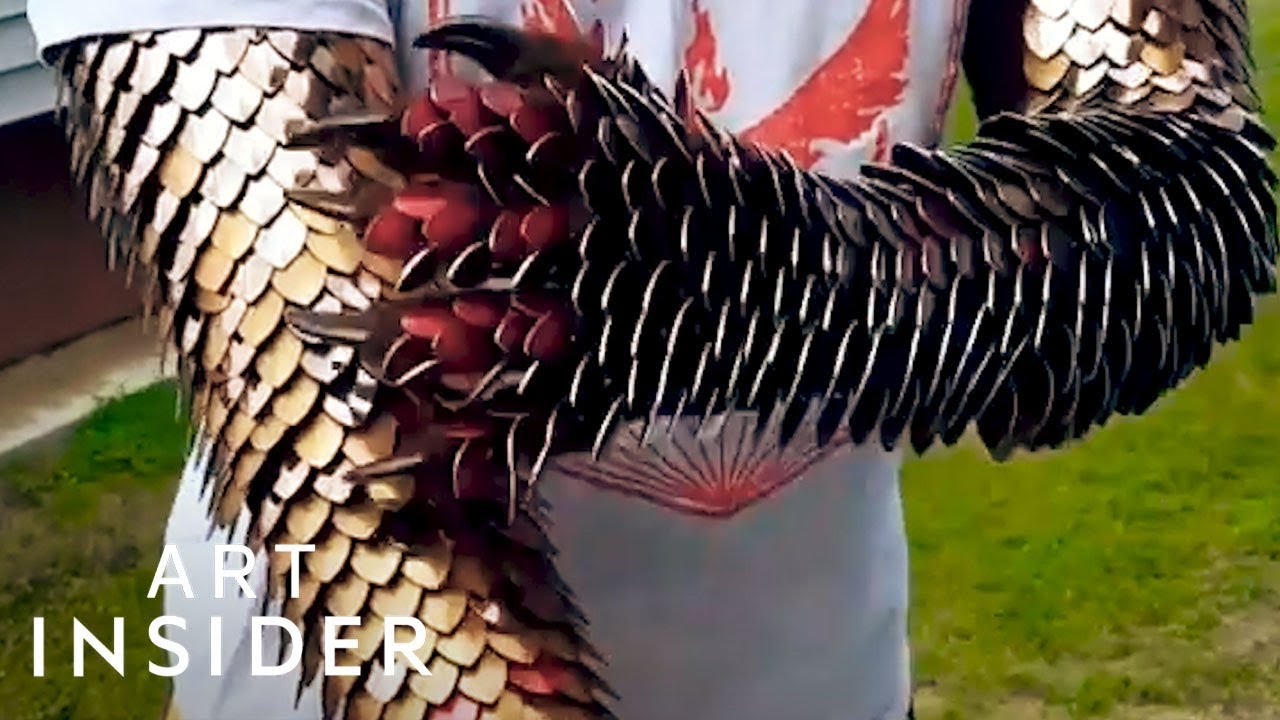This image appears to be a landscape-oriented screenshot, likely from a video, possibly a YouTube thumbnail, which includes the text "ART INSIDER" in all caps in white font in the bottom left corner. It is a close-up of a person wearing a stylized medieval-inspired suit of armor, focusing primarily on their torso and arms. The person is clad in a white fatigue adorned with an emblem, resembling a red-painted Phoenix, centrally positioned. The arms are covered in intricate, overlapping metal scales: gold in color, resembling small, heart-shaped plates for flexibility. The left arm is extended downward, while the right arm is bent across the chest, gripping the left arm. The fingertips on both hands transition from red scales to golden claws, emphasizing their elaborate design. This elaborate attire, which hints at cosplay, is set against a backdrop of a grass field, vividly highlighting the character's costume.